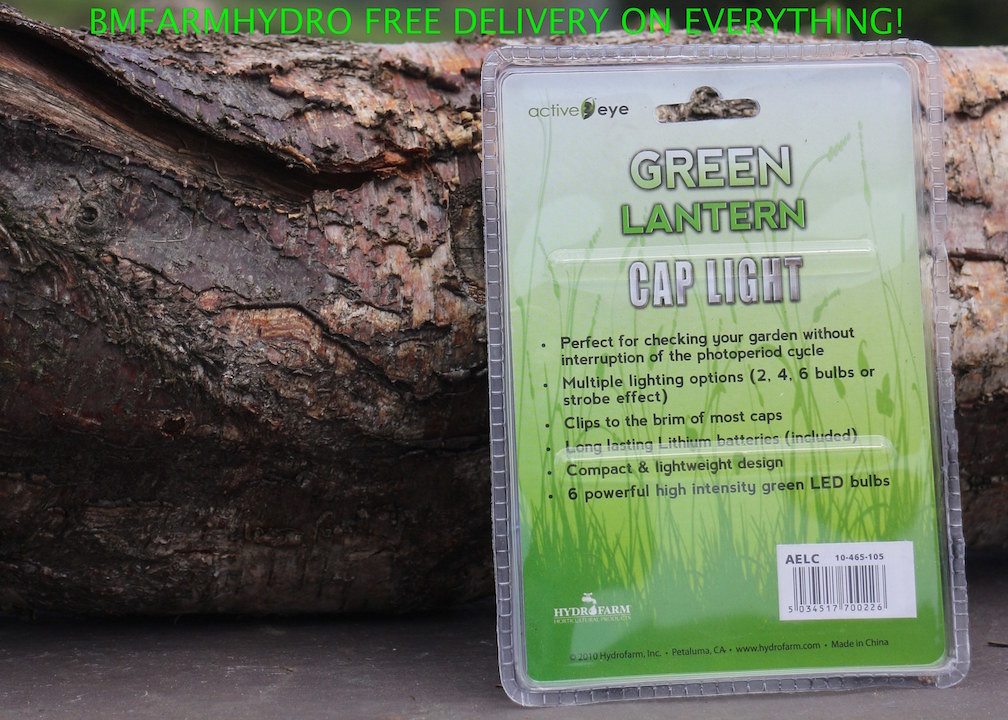The image features the ActiveEye Green Lantern Cap Light, presented in a heavily sealed plastic clamshell packaging. The prominent text on the package highlights its suitability for checking your garden without interrupting the photo period cycle, boasting multiple lighting options - 2, 4, or 6 bulbs, and a strobe effect. It can easily clip to the brim of most caps, powered by long-lasting lithium batteries, and features a compact and lightweight design with six high-intensity green LED bulbs. The packaging, set against a backdrop of black with a silhouette of tall grass and flowering stems, is propped up on a weathered, knotted log with orange highlights. Positioned in an outdoor setting and appearing to lean towards the center right of the frame, the image also advertises BM Farm Hydro’s offer of free delivery on everything, clearly conveyed at the top of the image. Surrounding hues include shades of brown, green, light green, gray, white, and black, reflecting an outdoor environment.